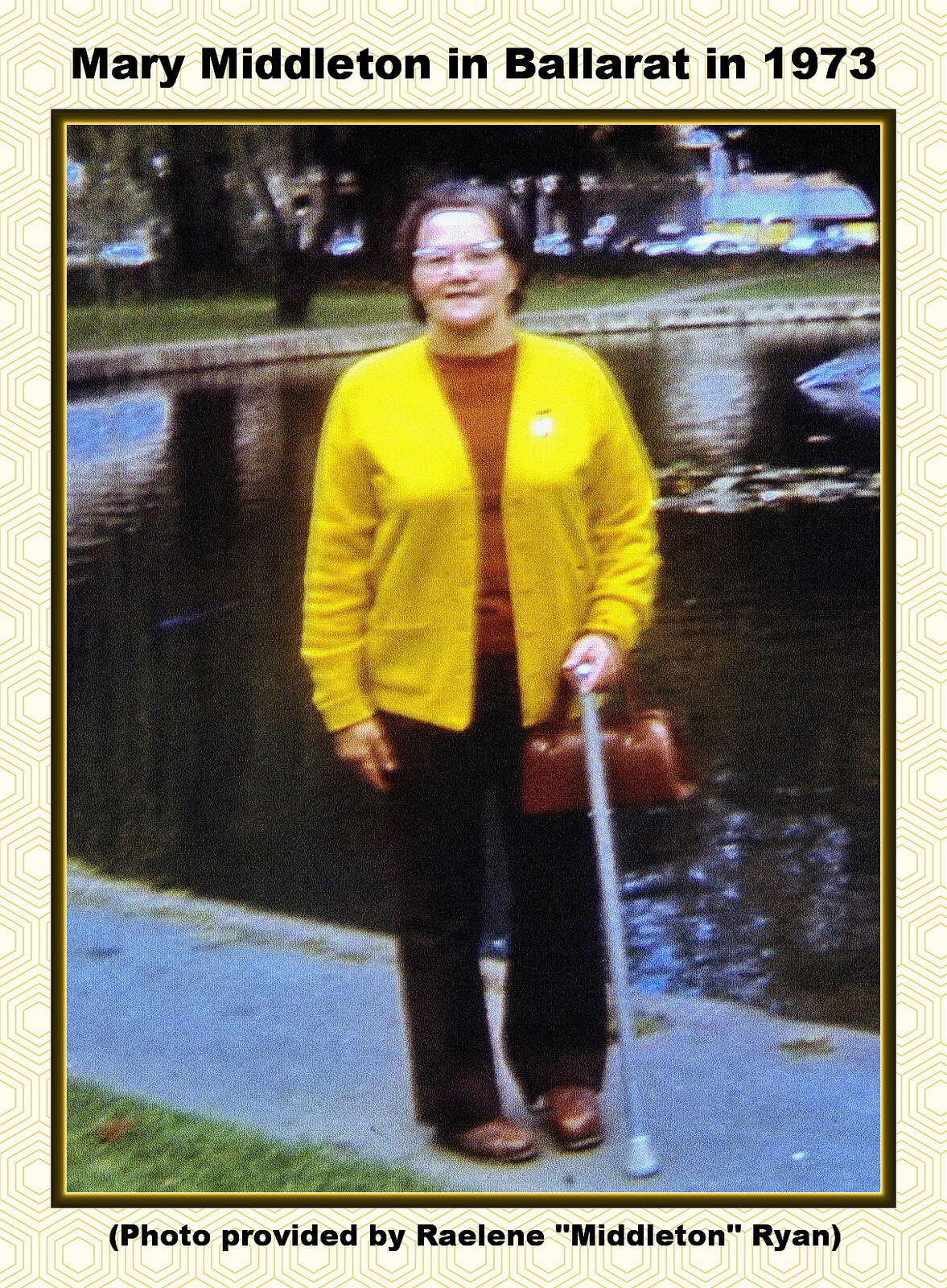The image depicts a grainy, faded photo from 1973 of an elderly Caucasian woman named Mary Middleton, taken in Ballarat. She stands on a sidewalk adjacent to a small, dark gray pond or fountain, with sun ripples and blue sky reflecting on the water. Behind her, there is a lawn, trees, and indistinct buildings. Mary has short to medium-length curly dark hair and wears glasses with a neutral expression. She is dressed in a yellow honeycomb-patterned blazer over an orange-brown blouse, black pants, and brown shoes. Over her left wrist, she carries a brown handbag and holds a gray cane in her left hand. The photo is framed with a yellow honeycomb border, and at the very top, in dark letters, it reads "Mary Middleton in Ballarat in 1973." Below the photo, in parentheses, it notes "Photo provided by Raylene ‘Middleton’ Ryan."